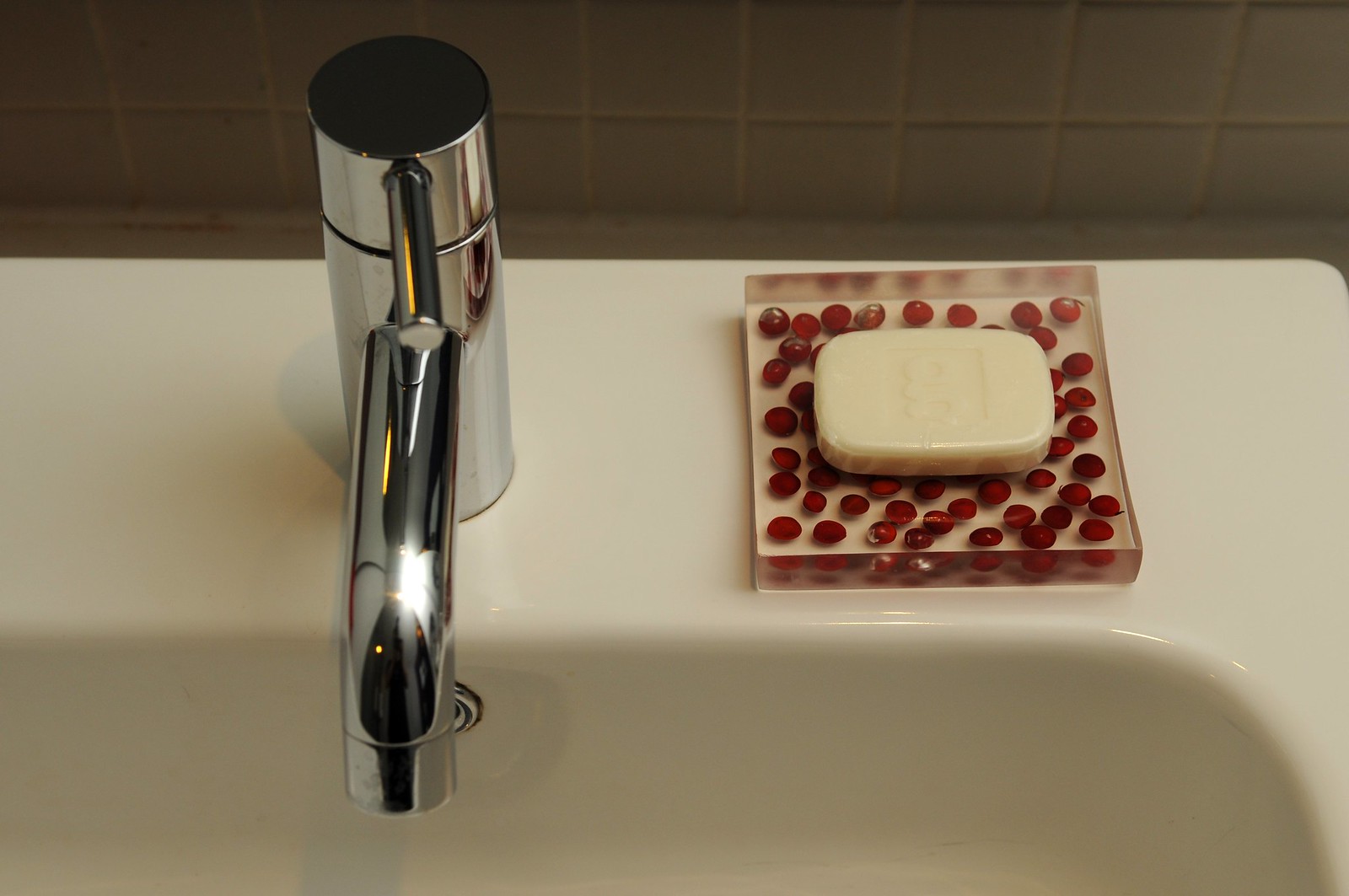This horizontal close-up photograph captures the corner of an almond-colored porcelain sink in a bathroom. The background features a small square brown tile wall, adding a rustic charm to the setting. The sink is accompanied by a simple stainless steel faucet, which has a rod-shaped, one-handle twist mechanism with a black cap on top. This handle serves to rotate the faucet for controlling the water flow. To the right of the sink is a clear acrylic soap dish, containing a single layer of red, circular, oblong objects, giving it a splash of color. Atop this soap dish lies an ivory-colored bar of soap, with an embossed label featuring a flower petal design inside a square, enhancing the cleanliness and minimalism of the scene.